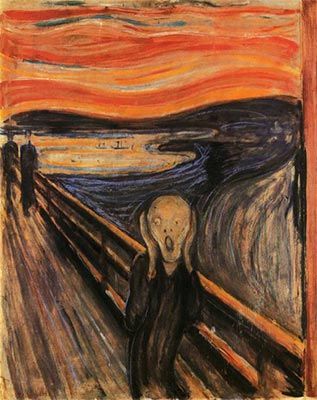The image depicts a cropped section of Edvard Munch's famous painting, "The Scream," recreated with what seems to be pastel or acrylic paint. Centered in the bottom of the image is a bald figure with a humanoid, skull-like head, a wide-open mouth forming an oval, and hands pressed to the sides of its face in an expression of intense alarm. The figure wears a black outfit and stands on a bridge, which extends toward the left side of the image, displaying its wooden frame in brown hues. Two silhouetted figures, dressed in black, are seen walking in the distance on the bridge. The background sky is a vibrant swirl of oranges, reds, and touches of green, rendered in curving horizontal stripes that create a striking and chaotic atmosphere. To the right side, a body of water, characterized by its blue and white scribbled appearance, intertwines with the dynamic scene, enhancing the painting’s sense of turmoil and emotional intensity.